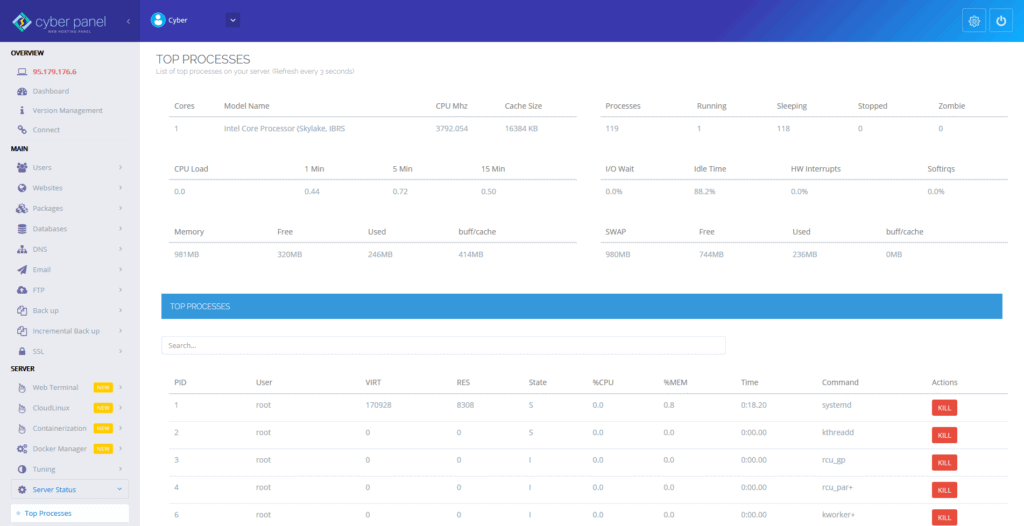The image appears to be a screenshot from a website interface. At the top, the website's name is prominently displayed, and there are sections labeled "Top Processes" and "Channels," though part of this area is obscured. On the left side, a navigation menu lists options such as "Overview," "Main," "Server," and "Top Processes." The upper part of the image includes a blue rectangle that transitions into a lighter, royal blue towards the right, where there are power and gear icons, presumably for settings and power functions.

The background below this header is primarily white. Centrally, there is another blue rectangle, lighter than the one above, adding a visual contrast. The main content area is organized into columns with headers including PID, User, Vert, Rest, State, % CPU, % MEM, Time, Command, and Actions. Each row in these columns is populated with data, and on the far right, there are five red "Kill" buttons, likely for terminating processes. This detailed layout suggests a process management interface, possibly for a server or application monitoring system.